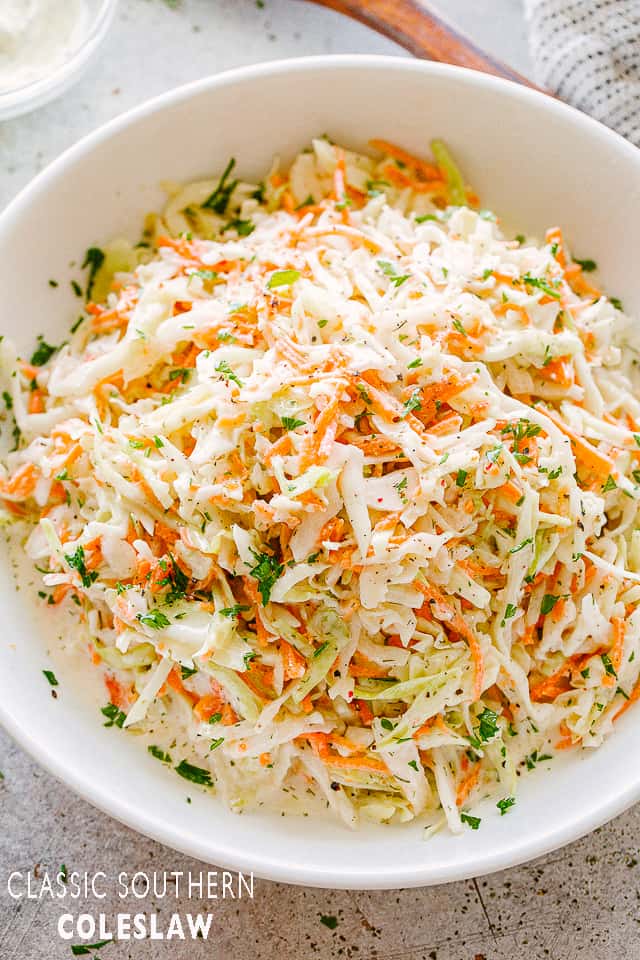In this photograph, titled "Classic Southern Coleslaw" as noted in white text at the bottom left, a generous, colorful bowl of coleslaw takes center stage. The coleslaw, contained in a large white bowl that appears to be either ceramic or plastic, features a vibrant mix of shredded cabbage, both green and white, orange carrots, and sprinkled green herbs. It also seems to be garnished with something resembling white grated cheese. 

The bowl sits on a white, speckled marble or granite surface, adding a touch of elegance to the composition. Towards the top of the image, an array of kitchen essentials can be seen, including the handle of a wooden spoon positioned from the top middle down to the right, resting beside a gray and white striped towel. Additionally, a bowl with a white substance and a glass plate make subtle appearances in the background, adding depth and context to the scene. The entire photograph, bathed in natural light, captures the rustic charm and aesthetic appeal of this classic Southern dish.